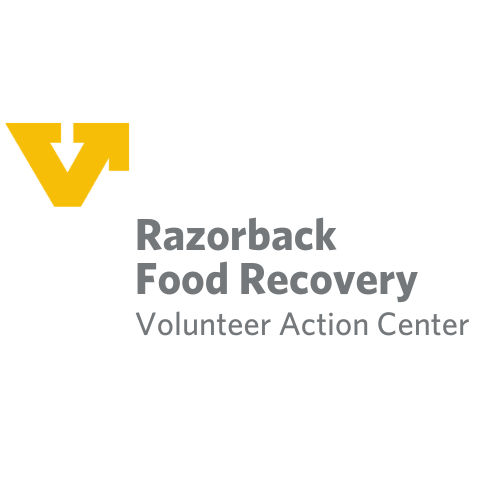The image is a digital poster featuring a distinct logo and text on a plain white background. At the upper left corner, there is a dynamic, almost triangular logo in a yellowish-gold color. The logo is designed as the letter 'V,' where the right arm transitions into an arrow pointing upwards and to the right, suggesting motion and action. Embedded within the V is a downward-pointing white arrow, adding depth to the design. To the bottom right of the logo, there is gray text arranged neatly in three lines. The first two lines, "Razorback" and "Food Recovery," are bolded, while the third line, "Volunteer Action Center," is in regular font. All elements combined convey a sense of organized volunteerism and active engagement.